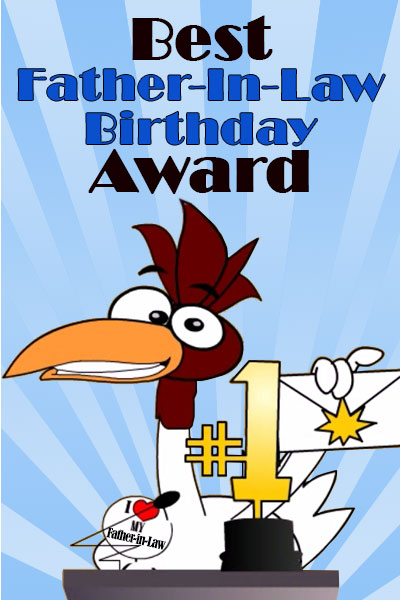The image is a vertical, rectangular card with a vibrant blue background featuring sunbeam patterns in varying shades of blue, radiating from the bottom towards the edges. At the top center, the text reads "Best" in bold black letters, followed by "Father-in-Law Birthday" in dark blue, and "Award" in black. Below the text stands a whimsical chicken with a brown head and white body, characterized by large white eyes with black specks, and a quirky smile that shows its teeth. The chicken has an orange beak pointing to the left and is holding a white envelope sealed with a gold star in its three claws. Adorning its chest is a pin that reads "I ♡ My Father-in-Law." The chicken is positioned behind a gray podium with a black, zigzag-shaped microphone wire extending from it. On the podium rests a golden trophy inscribed with "Number One."